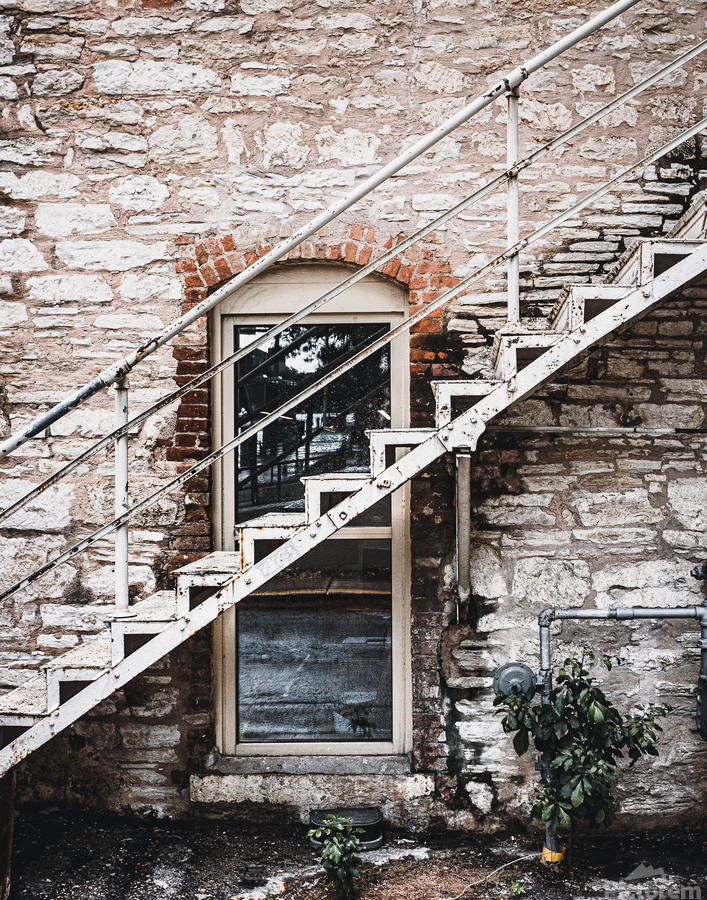This detailed photograph captures the exterior of an old, stone building featuring a prominent arched window at ground level. The window has two panes of glass and is topped with a curved arch of red bricks. A worn, white-painted iron staircase diagonally traverses the image from the bottom left near the window to the top right, leading to an unseen upper level. The staircase, with three protective railings, fastens to the wall to the right of the window. The juxtaposition of the modern glass door, surrounded by red bricks, adds an element of contrast against the building's historical stone facade. The scene feels slightly ironic due to the outdated architecture clashing with the contemporary door and the awkward placement of the staircase, which intrudes upon the window.